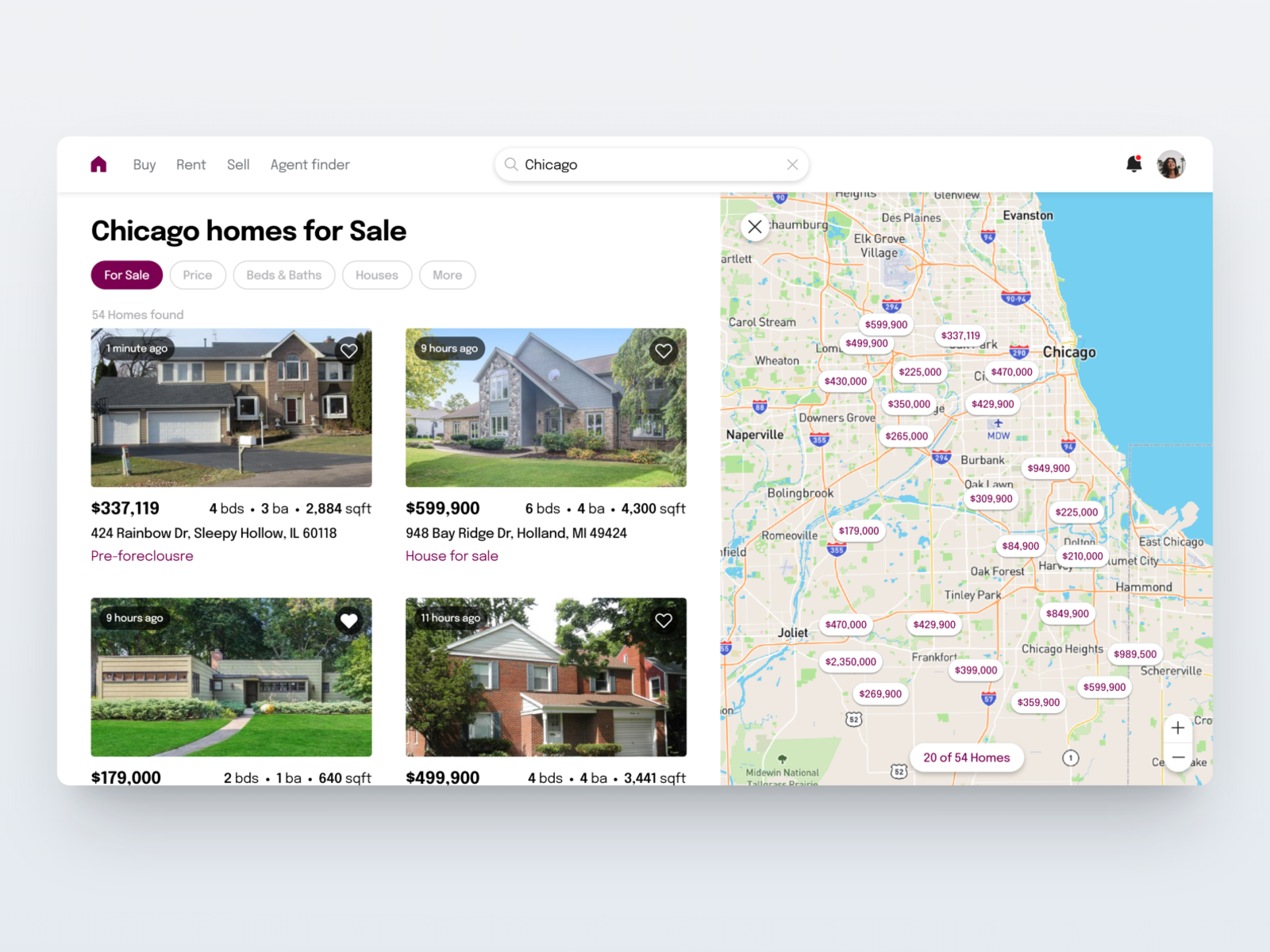A screenshot from a real estate website is displayed in a large gray frame. Centrally positioned is the website interface featuring a header with a distinctive plum-colored house icon. Below the icon are navigational options including "Buy," "Rent," "Sell," and "Agent Finder," all in a muted gray tone. A prominent white search box displays "Chicago" in gray text. Adjacent to it are icons: a gray bell notification with a red dot and a circular user profile picture.

The main heading in black reads "Chicago homes for sale," followed by a plum-colored circle labeled "For Sale." Further filters listed in gray are "Price," "Beds & Baths," "Houses," and "More."

A series of property listings feature images and descriptive text below. The first property shows a two-story, tan-colored house with white windows, priced at $337,119. It offers 4 beds, 3 baths, and covers 2,884 square feet, located at 424 Rainbow Drive, Sleepy Hollow, Illinois, 60118, marked "Pre-Foreclosure" in purple.

The second listing is a tan and gray, two-story home priced at $599,900, offering 6 beds, 4 baths, and 4,300 square feet, located at 948 Bay Ridge Drive, Holland, Michigan, 49424, noted as "House for Sale" in purple.

The third property, an olive-toned house priced at $179,000, features 2 beds, 1 bath, and 640 square feet, though the address text is partially cut off.

The final listing showcases a two-story brick house with gray shutters, priced at $499,900, offering 4 beds, 4 baths, and 3,441 square feet.

On the right side of the image, a map of the Chicago area is displayed, highlighting areas including Evanston, Chicago, Naperville, and Joliet. The map is dotted with white circles containing plum-colored property prices, ranging from $200,000 to over $2 million. The bottom text indicates "20 of 54 homes" displayed in a combination of white and plum text.